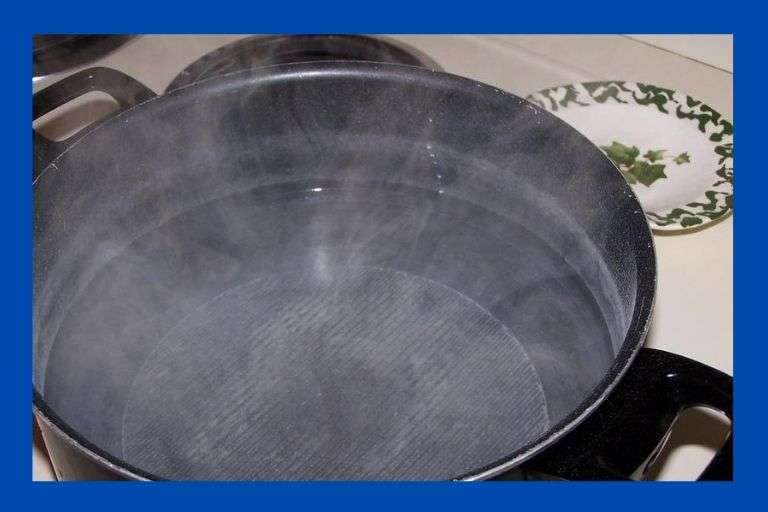In this detailed image, we see a scene set in a personal kitchen. The focus is on a large, silver pot with black plastic handles on a white stovetop situated toward the bottom left and extending towards the center of the frame. The pot contains clear water that is beginning to steam, suggesting it is heating up but not yet boiling. Surrounding the pot, we notice various colors including blue, white, tan, green, black, and different shades of gray. A distinct thick blue border frames the entire image. In the upper right corner, there is a white porcelain plate featuring a green leaf design in the center with a matching leaf pattern around the edges. Near the top left of the image, another unused stovetop burner with a black coil is visible. The background primarily shows a white surface, enhancing the focus on the kitchen elements and the live cooking activity.